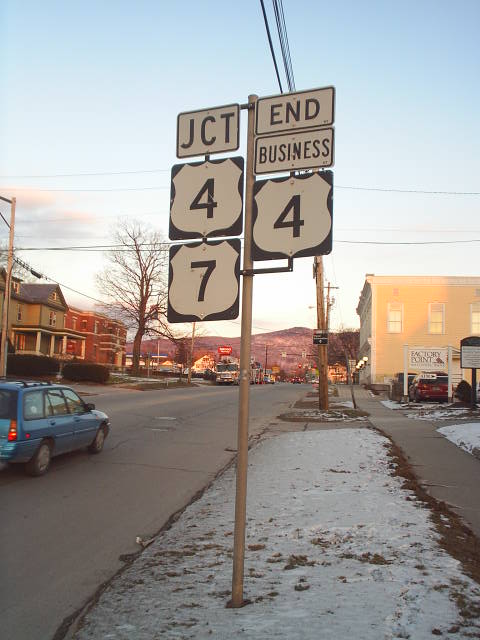The image depicts a busy urban intersection dominated by a variety of street signs and a lively backdrop. Central to the photo is a patch of grass, bordered on the right by a sidewalk, and in the background, a white building with three visible windows. A prominently placed sign reads "Factory Point," with a red van parked just behind it in a small parking lot.

In the foreground, a tall silver pole displays multiple street signs. The top sign is labeled "JCT" in black lettering within a white box, followed by the numbers "4" and "7" on separate signs beneath it. Another sign on the same pole reads "END BUSINESS 4." Overhead, electrical power lines are connected to the poles.

To the left of the pole and signs, the street stretches out where a blue station wagon can be seen driving. Across this street, two distinct buildings stand out: one painted green and the other composed of red brick, the latter featuring prominent white pillars. Further down the street, a parked fire truck is visible, suggesting an emergency presence or a routine visit.

A gas station with a blue and white roof can be seen to the left, marked by a partially visible sign. An adjacent red and white sign adds a pop of color to the scene, although the text is not legible. This detailed and bustling cityscape encapsulates a snapshot of everyday urban life, filled with movement and various architectural features.